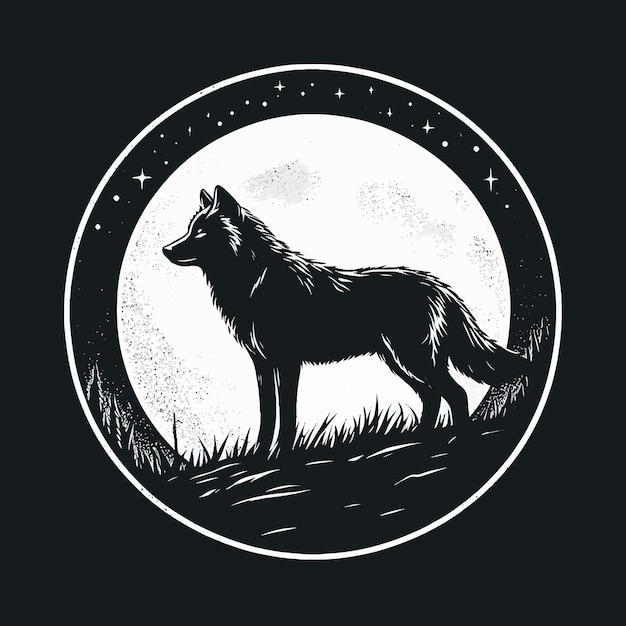The image features a black background with a square border enclosing a white circle. Inside the white circle is another black circle adorned with twinkling stars at the top, creating a night sky effect. Central to the composition, a large, bright full moon illuminates the scene. Superimposed on the moon is a detailed silhouette of a wolf, standing alert on some blades of grass. The wolf, primarily black with whitish highlights suggesting moonlight shadows, gazes into the distance. Surrounding the moon at the edges of the black circle are the faint silhouettes of trees, enhancing the nocturnal ambiance. The entire image is rendered in black and white, emphasizing the stark contrast and the serene, ethereal quality of the moonlit night.